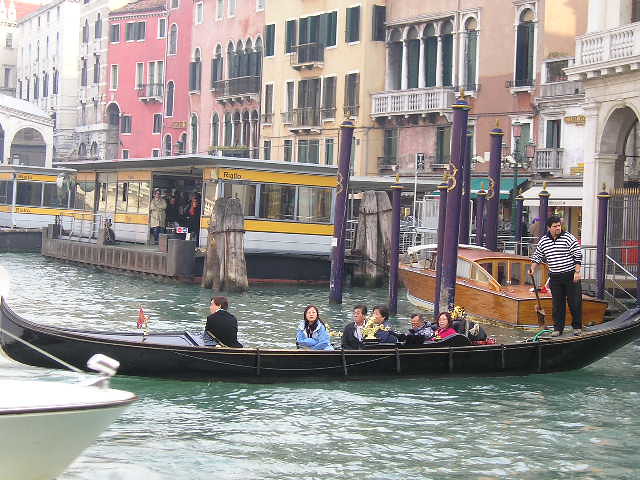In this vibrant, color photograph set in Venice, Italy, a black gondola glides along a green, gently undulating waterway. The gondolier, donning black trousers and a black-and-white striped shirt, is standing on the right side of the boat, gazing thoughtfully into the distance while grasping a punting stick. The gondola, slightly cut off at the edges of the frame, is occupied by a diverse group of tourists, including a woman in a blue jacket, two Asian individuals dressed in black jackets, an Asian couple with one in a pink jacket and the other in blue, and someone sitting at the front. Behind the boat, other vessels can be seen navigating the waterway.

The backdrop features a row of closely-packed, colorful buildings on the right side that fade into the distance on the left. These buildings are painted in a palette of rich hues including white, pale yellow, a faded salmon pink, a vivid pink, and a burnt orange. Additionally, there is a shelter with a flat roof and white and yellow sides adorned with black barber-pole-styled posts nearby, indicating it might be a docking area for other gondola rides or a waterside restaurant. The scene is quintessentially Venetian, capturing the charm and bustling activity along the Grand Canal amidst its iconic, picturesque architecture.